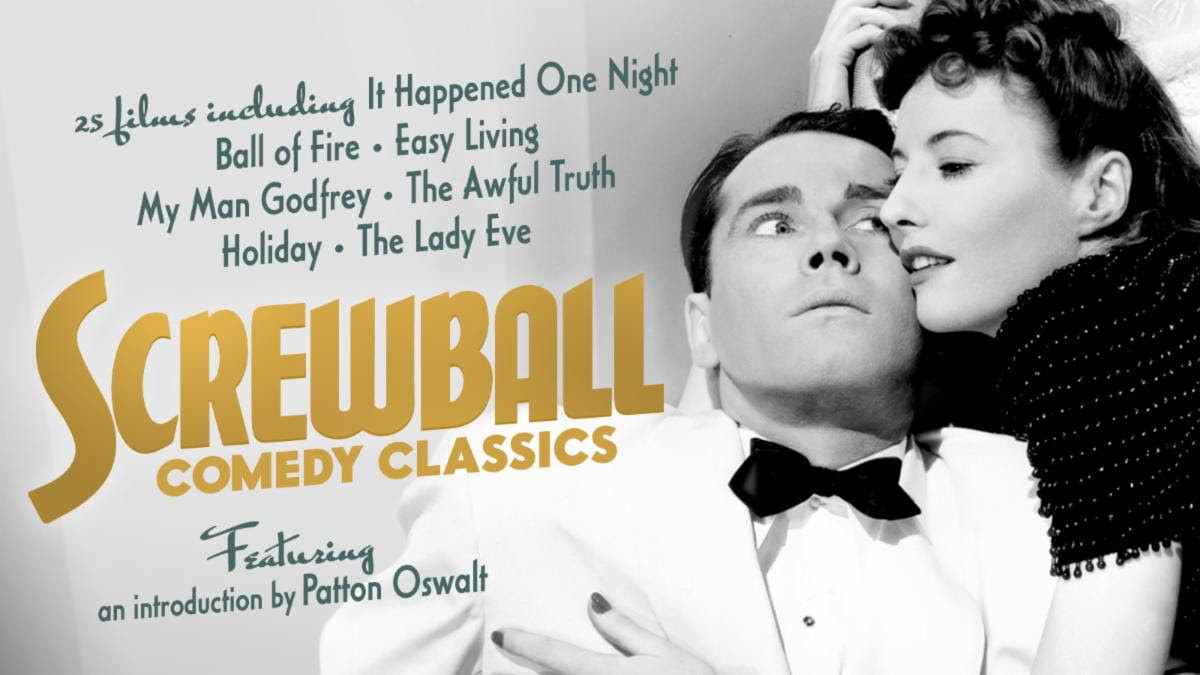The image appears to be a black and white horizontal movie poster. It features a woman dressed in an evening gown, though only her shoulder is visible. She is a white woman with dark, wavy hair, and she's intimately holding a white man with short dark hair who is dressed in a white tuxedo with a black bow tie. The woman looks caring while the man appears alarmed or shocked. On the left side of the image, aqua blue text lists several films: "25 films including It Happened One Night, Ball of Fire, Easy Living, My Man Godfrey, The Awful Truth, Holiday, The Lady Eve." Beneath this, in gold text, it reads "Screwball Comedy Classics," and following that, more aqua blue text says "featuring an introduction by Patton Oswalt."